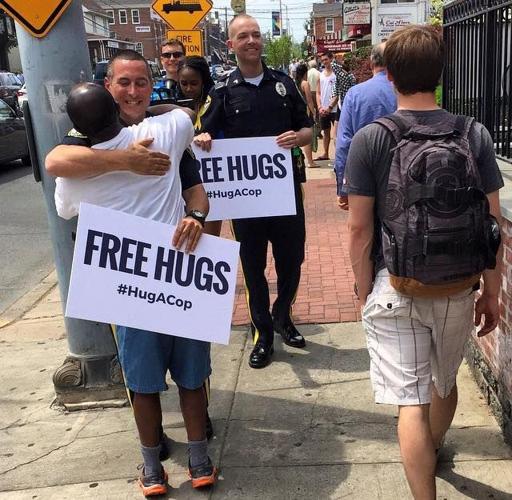In the photograph, taken outdoors during the daytime in what appears to be an East Coast city like Philadelphia, two police officers dressed in dark blue uniforms are engaging warmly with the public. They both hold white signs that read "Free Hugs" and "Hug a Cop." One officer is hugging a black man who is dressed in a white t-shirt, knee-length denim shorts, and gray shoes. The second officer stands to the side, smiling, and holding a similar sign. Nearby, another person, likely a passerby, is dressed in a gray shirt, cream-colored shorts, and carries a gray Mark Echo backpack. The scene is set on an urban street with a sidewalk filled with friendly pedestrians, one of whom appears to be recording the interaction, suggesting a casual and welcoming atmosphere.